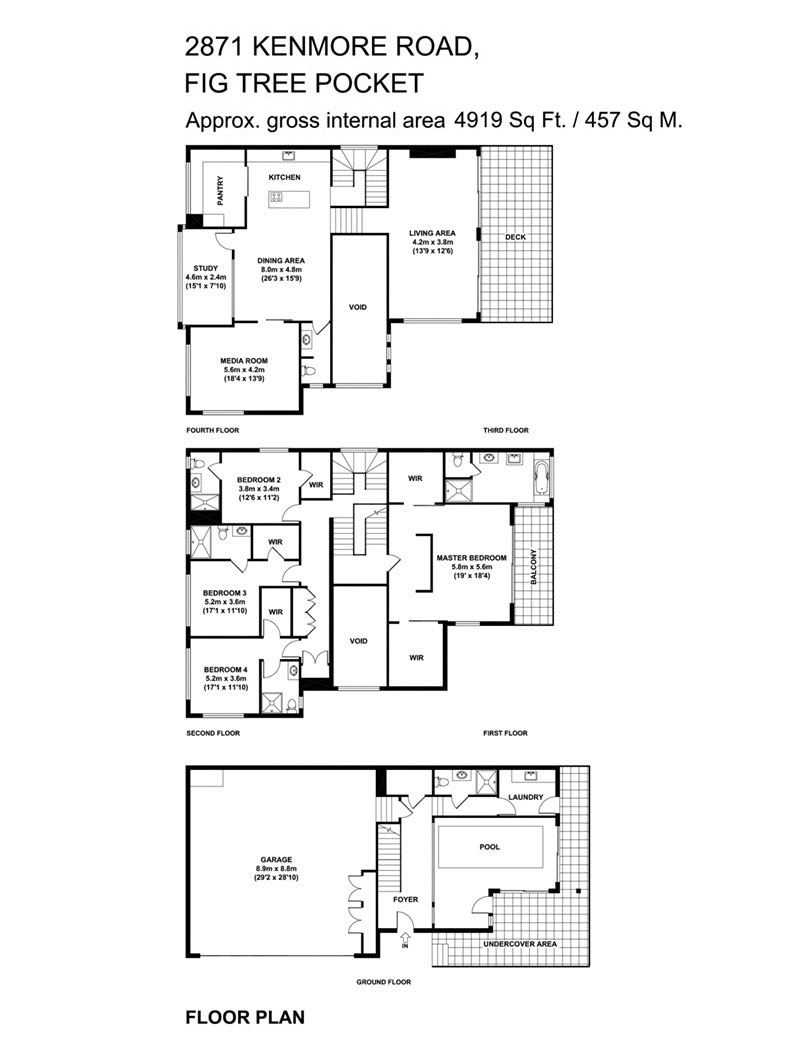The image depicts a detailed, black-and-white floor plan of a three-story house located at 2871 Kilmore Road, Fig Tree Pocket. At the top of the graphic, bold black text states, "2871 Kilmore Road, Fig Tree Pocket," followed by smaller text that reads "approximately Gross Internal Area 4,919 square feet / 457 square meters." The floor plan is divided into three sections, each representing a different floor of the house. The ground floor features the garage, foyer, laundry area, an uncovered outdoor space, and a pool. The second floor showcases three regular bedrooms, one master bedroom, and an adjacent bathroom. The top floor consists of communal spaces, including a living area, dining area, study, and media room. The layout is clearly delineated in black and white, with the overall blueprint occupying the central portion of the image, and large text at the bottom reads "floor plan," denoting its purpose as a design schematic for a residential property.